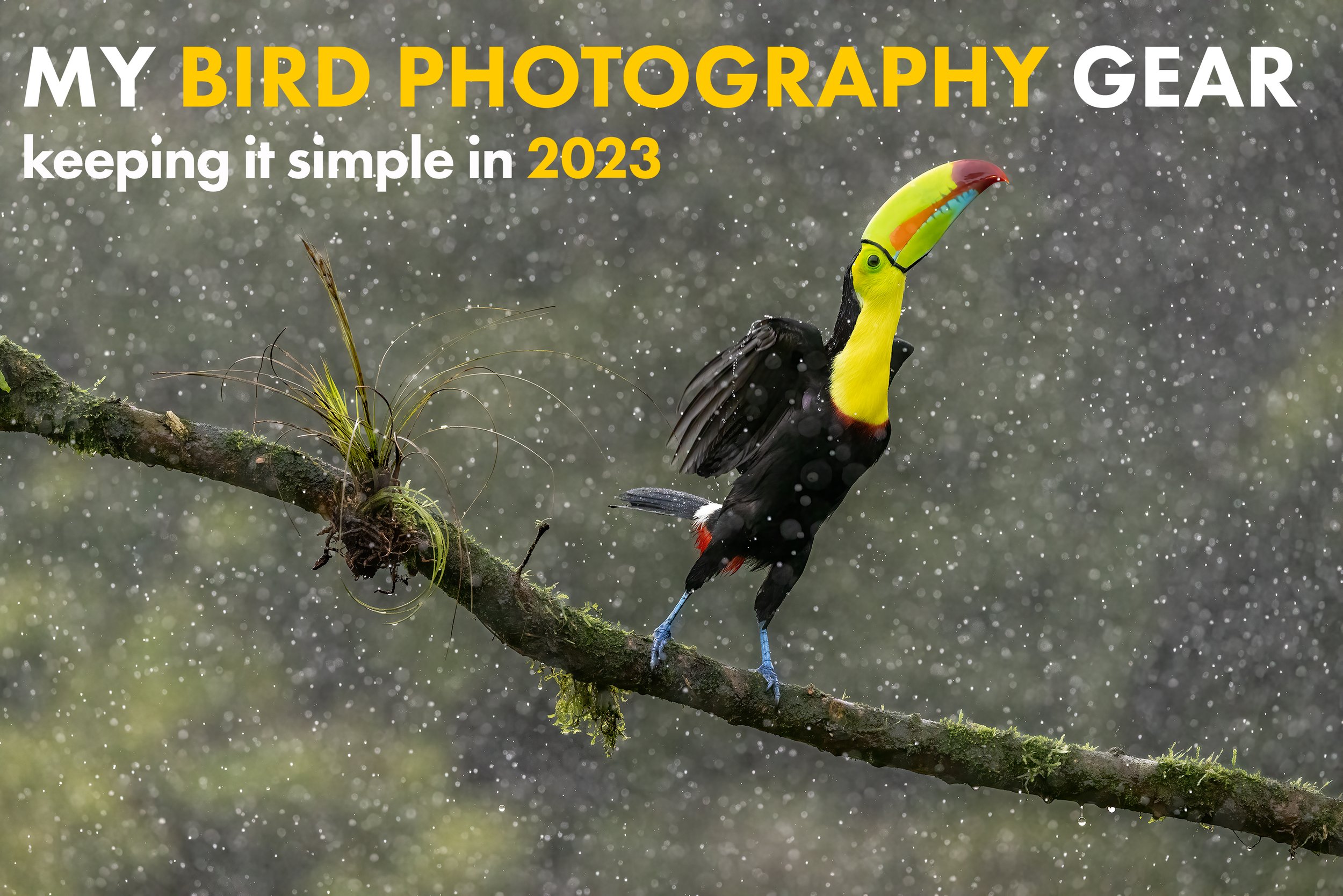This horizontal rectangular photograph captures an unusual and vibrant bird perched on a mostly bare tree branch that extends from the lower right to the center of the left side of the image. The bird, which resembles a parrot, stands almost straight up, with its enormous, multicolored beak pointing upward. It features a magnificent array of colors: striking blue feet, a predominantly black body and wings, a yellow head and neck, black feathers, and a unique tail marked with a red hue and a white band. The background is an unfocused, brownish color, possibly indicating rain or a fuzzy natural setting. Above the bird, text reads: "MY BIRD PHOTOGRAPHY GEAR, keeping it simple in 2023," with variations in capitalization and colors for emphasis. The bird's vivid and varied colors, combined with its unusual posture and the simplistic natural setting, create a compelling and visually captivating scene.